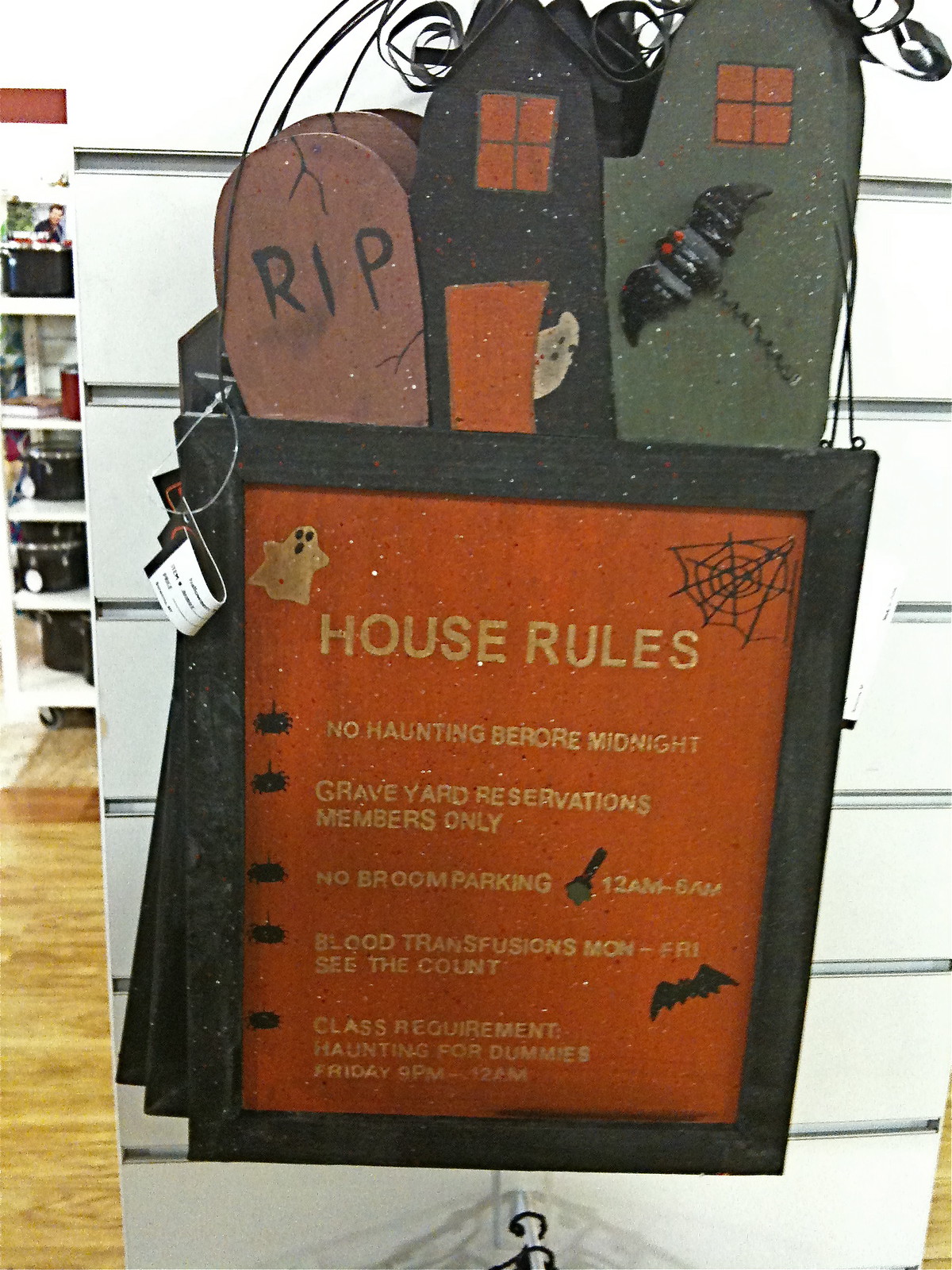The image depicts a Halloween-themed house rules sign, designed with a whimsical touch. Set against an orange background, the rules are written in gold, likely due to a shortage of white ink. The sign features a black border adorned with thematic decorations: at the top, a grey stone inscribed with "R.I.P.," a black house with red windows and door, and a grey house with a bat affixed to a red window. On the left-hand side, there's an illustration of a ghost, while the right-hand corner features a cobweb design. Each rule is accompanied by a small spider graphic. The playful and spooky rules outlined are: "No haunting before midnight," "Graveyard reservations members only," "No broom parking 12 a.m. to 6 a.m.," "Blood transfusions Monday to Friday, see the Count," and for "Class requirements, 'Haunting for Dummies,' Friday 9 p.m. to 12 a.m." This sign combines both aesthetic and humorous elements, making it a perfect Halloween décor piece.